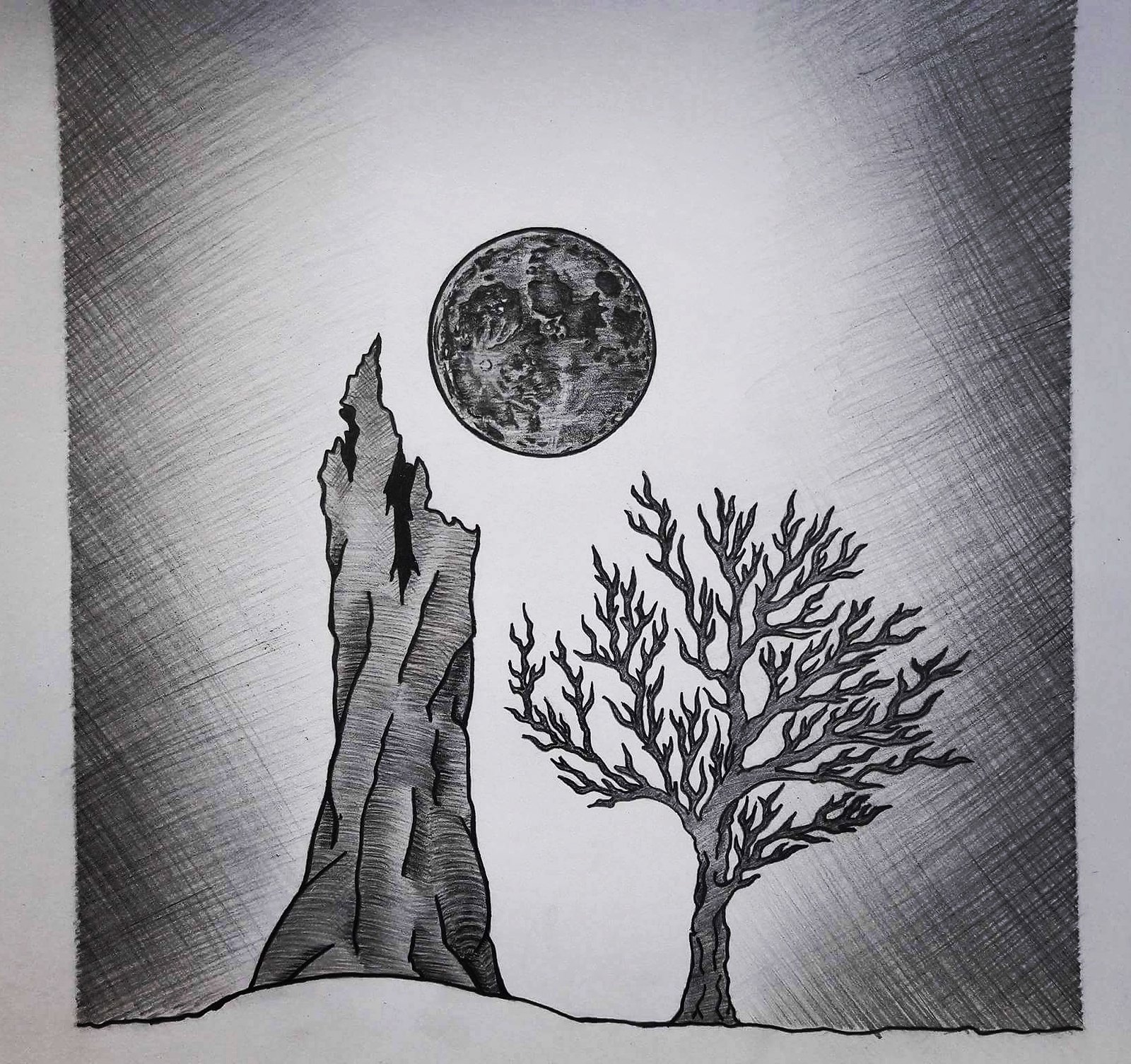The image is a highly detailed, digitally-created black and white drawing on a white background. It showcases a desolate scene with complex shading and texture work. At the center, a heavily cratered moon is depicted in dark gray, almost light black hues, surrounded by a gradient from white to black, creating a dramatic contrast. Below the moon to the left, there stands a tall, broken-off tree trunk with no top, characterized by its sharp points and intricate texture. Adjacent to this trunk, a dead tree with numerous smaller branches, each about an inch long, adds to the barren landscape. The edges of the drawing feature a hatch pattern that darkens towards the periphery, enhancing the focus on the central elements. The ground is slightly uneven, adding to the rough and raw nature of the composition.